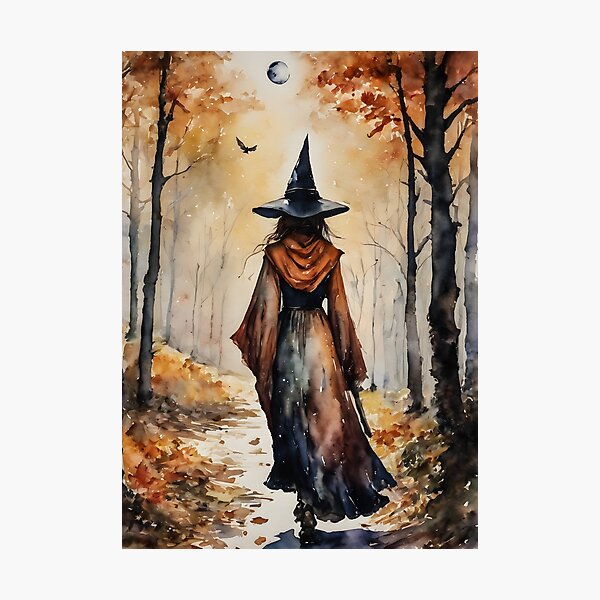Under the pale, eerie light of a full moon, a witch walks along a gravel path in the midst of an autumnal forest. Trees, painted in deep blacks and oranges, flank either side of her with their bare branches, while fallen leaves blanket the ground, enhancing the season's ambiance. The witch, viewed from behind, dons a wide-brimmed, sharp-pointed hat and a flowing gown that transitions from earthy browns at the top to inky black towards the bottom. Her dress, featuring rust-colored sleeves and a tan-gray accents, is complemented by a shawl draped over her back. A black bird soars above her, silhouetted against the moon, adding to the mystical atmosphere. The intricate details of the scene— from the witch's pointed hat and flowing gown to the detailed depiction of the fall forest— suggest it is a painted artwork, capturing the haunting beauty of a witch’s solitary journey under the moonlight.